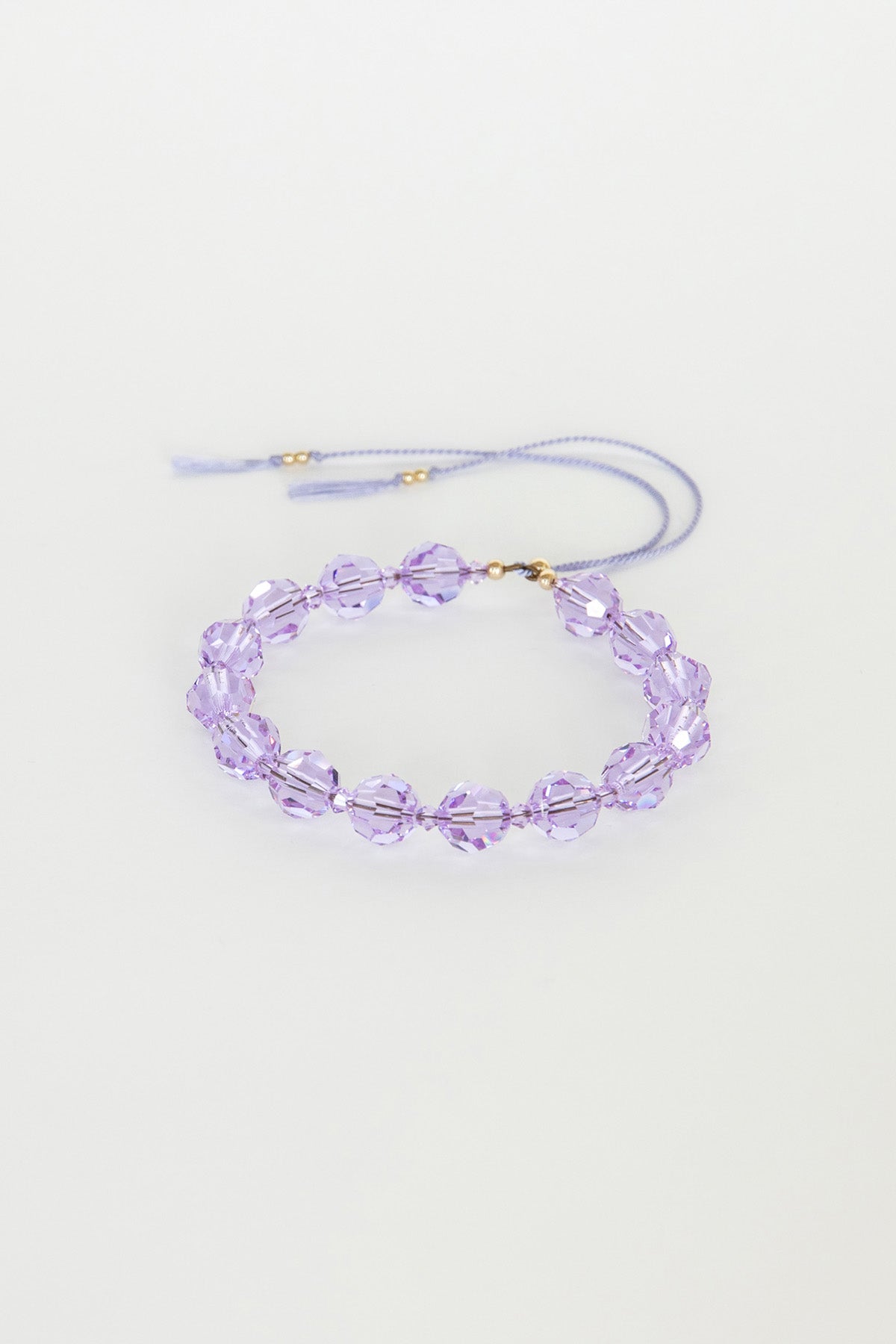The image features a delicate bead bracelet composed of translucent, light purple crystal beads, each approximately the size of peas. These beads form a circular arrangement, strung together on a thread that is secured by a gold clasp. Attached to the clasp are two additional purple strings, each terminating with a gold bead. The bracelet is positioned vertically, lying flat against a grayish background, creating a subtle contrast and highlighting the shiny, glass-like quality of the beads.